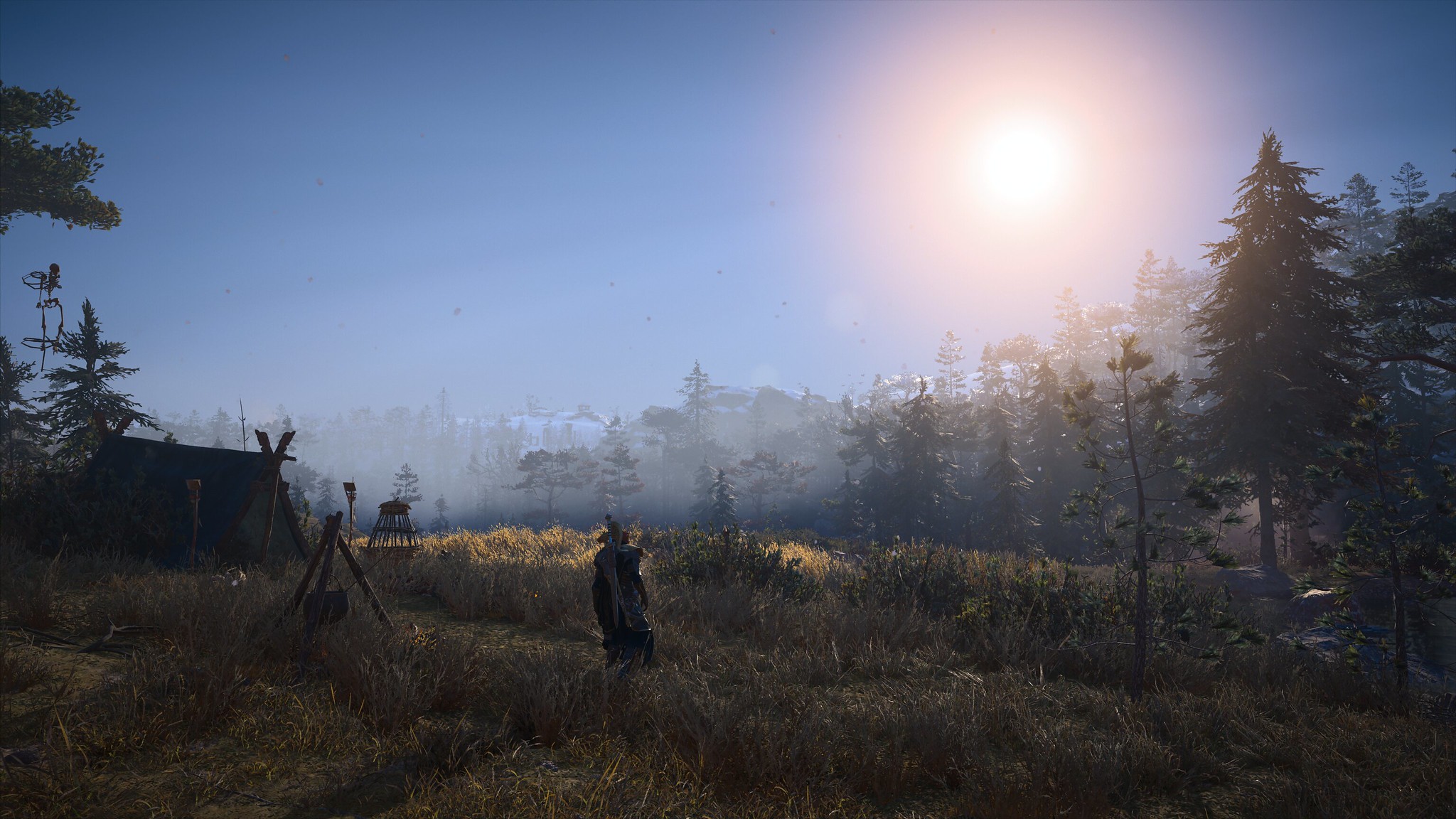A mesmerizing outdoor landscape photograph captures the early hours of dawn or dusk, evidenced by the radiant sun piercing through a delicate, hazy fog. The scene unfolds in a serene rural setting, devoid of human presence but abundant in natural and rustic elements. Dominating the foreground is a sprawling field bordered by dense clusters of trees. In the distance, amid the fog-obscured horizon, faint silhouettes emerge, suggesting the presence of distant buildings or possibly mountaintops.

To the left of the image, nestled within overgrown vegetation, stands a triangular-shaped tent or dwelling, evoking a sense of solitude and simplicity. Nearby, a tripod structure supports a kettle, implying the remnants of a recent outdoor cooking session. Adding to the rustic charm, another indistinct figure, possibly a scarecrow, lurks within the dimly lit environment, its features obscured by the interplay of shadows and fog. The overall composition, bathed in the ethereal light filtering through the mist, evokes a timeless and tranquil pastoral morning.